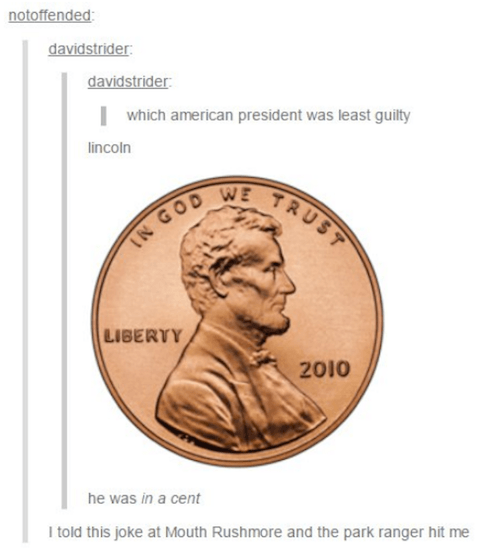The image is a humorous Tumblr thread centered around a photoshopped infographic of a copper-colored U.S. penny, featuring the front side with a side profile of Abraham Lincoln, and inscribed with "In God We Trust," "Liberty," and the year "2010." The original post by David Strider poses the question, "Which American President was least guilty?" and cleverly answers "Lincoln," followed by the pun explanation, "He was in a cent," alluding to the penny. Below the image of the penny, the user "not offended" adds a follow-up response: "I told this joke at Mount Rushmore and the park ranger hit me." The interaction captures a playful exchange of wordplay and humor between the two users.